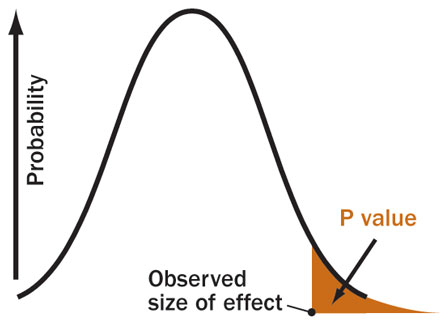This image is a detailed color graph featuring a prominent upward-pointing arrow on the left side labeled "Probability". The main focus is a curve resembling a bell shape that rises and then falls, visually representing the relationship between probability and the observed size of effect. At the base of this curve, an area is highlighted in orange, indicating the p-value. On the right-hand tail of this curve, both the p-value and the observed size of effect are marked, with the latter being specifically noted at the bottom. A small dot with a line connecting to the term "observed size of effect" underscores this point on the graph. The p-value label, also in orange, directs attention to the specific orange-highlighted section of the curve.